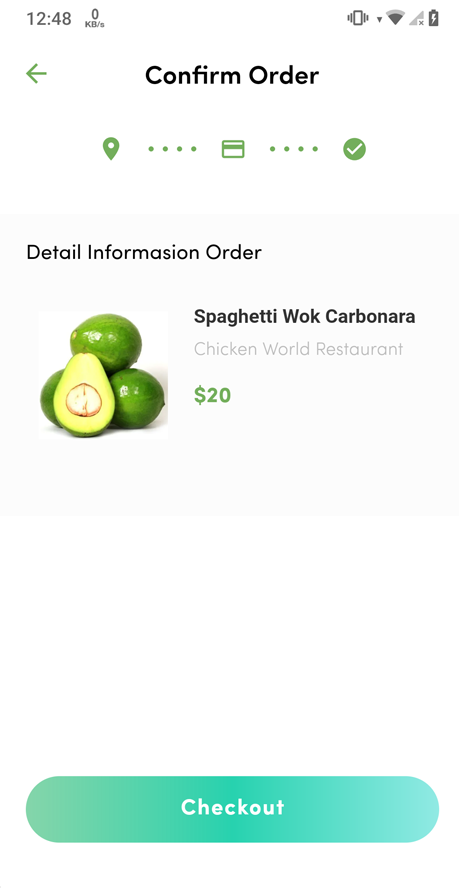The image is a screenshot from a mobile website. The top section features a status bar against a white background with dark gray text. It indicates the time "12:48" and displays "0 KB/s" alongside icons for a vibrating phone, a downward arrow, WiFi signal, cellular signal with an "X" (indicating no signal), and a battery with a light bulb icon inside.

On the left side below the status bar, there is a lime green left arrow. Prominently in the center is a bold, black text reading "Confirm Order" with capital letters "C" and "L". Below this, there is a green location icon followed by four dots in sequence. Next to the dots is a square intersected by a dark green line and four additional dots. Following that is a green circle containing a white checkmark.

Further down, there is a section titled "Detail Information Order," although "Information" is misspelled as "Informasion." Underneath, the text lists the items "Spaghetti Wok Carbonara" and "Chicken World Restaurant," with "SWAOK" mentioned, likely as an abbreviation or code. To the left of this text is a small square featuring three avocado icons and a price of "$20."

At the bottom of the screenshot, there is a teal green banner with the text "Check Out" in white.